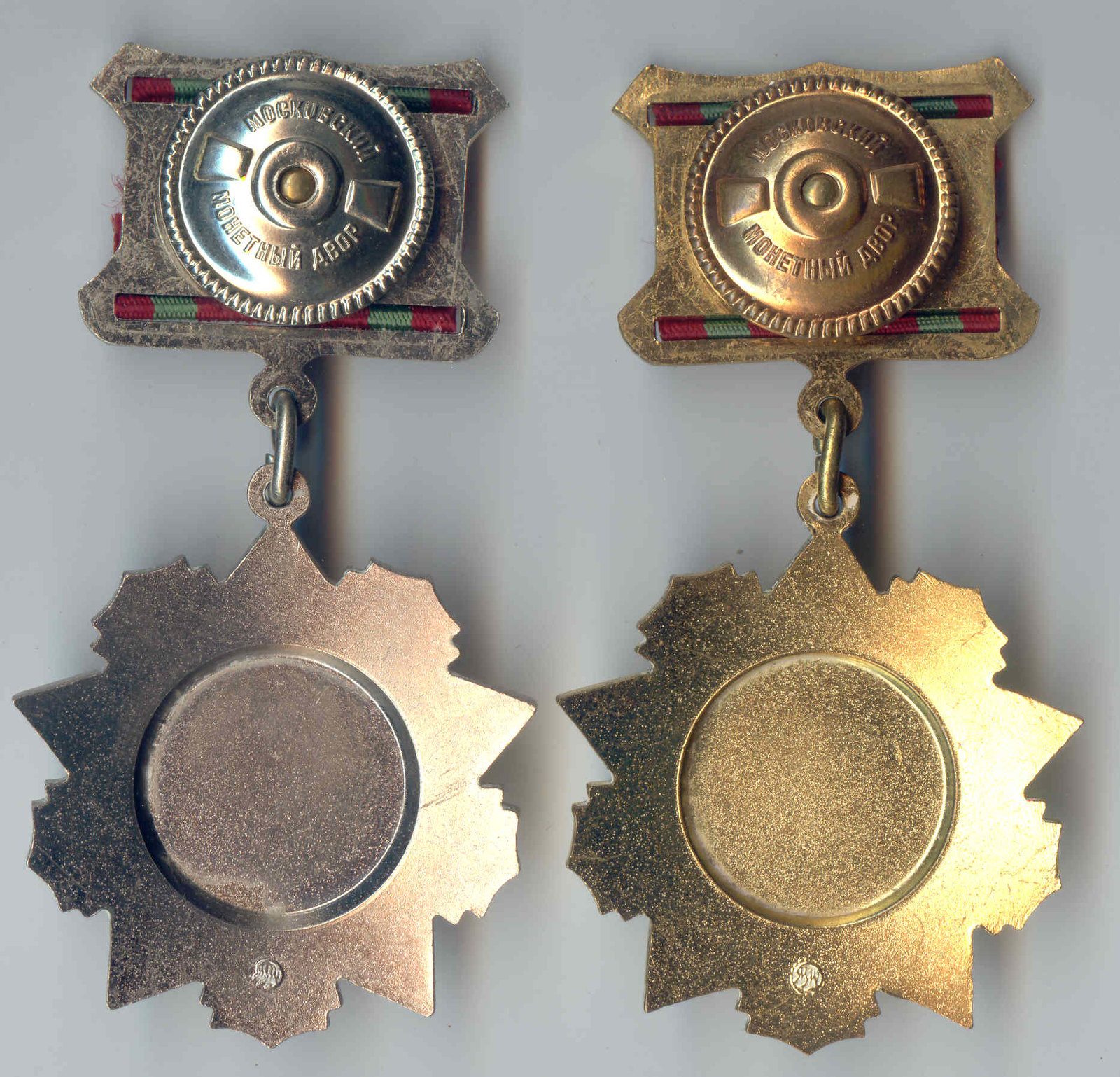This large square picture against a solid gray background showcases two distinct medals adorned with intricate designs and foreign script. The medal on the left features a blend of gold and silver hues, distinguished by its rectangular-shaped backing with a circular gold center. It has an elaborate design that includes a green and red cord threading through the rectangular part and a chain link connecting to a larger, irregularly edged medallion that appears partly brown and partly gold. On the right, the second medal mirrors the design of the first but leans more towards a dominant gold color. This medal also displays the same foreign writing at the top, with a circular metalpiece against the rectangular backing, transitioning through a single chain link to another distinctly shaped medallion at the bottom, completing the set in an eye-catching manner.